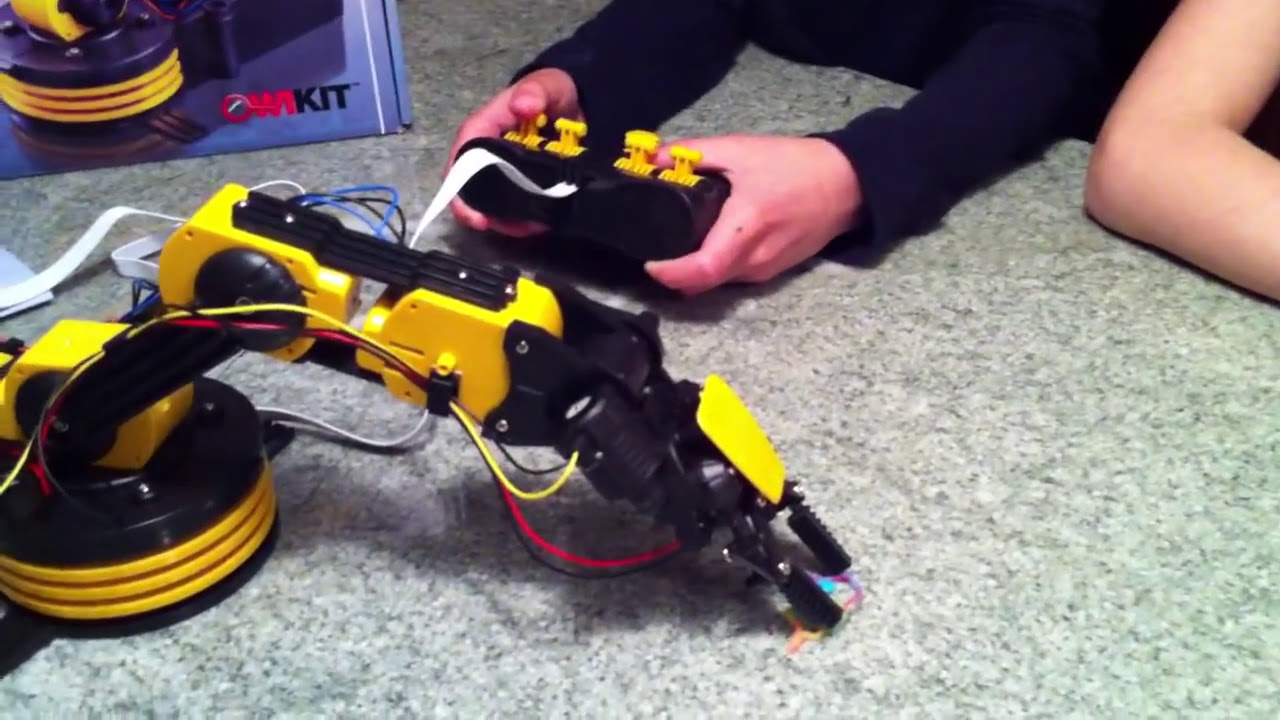The image features a detailed scene of a robotics kit known as an OWI kit, operated by two young individuals. One person, wearing a long-sleeved black shirt with visible forearms and hands, is positioned at the top right of the image, holding a black controller. This controller has four distinctive yellow joysticks and a white cable extending from its top. To the right of this person is another individual, whose bare arm and elbow rest on a gray marbled surface, appearing to observe the activity.

At the center of the scene is a yellow and black robotic arm, equipped with two joints and ending in two black pinchers. This robotic arm is operating various servos to pick up objects. Several yellow, red, and black wires run along the arm, emphasizing its intricate electronic structure. The arm is anchored to a rounded base adorned with three yellow rings, providing stable support for the device.

Overall, the image showcases a sophisticated electronics kit designed to teach young enthusiasts about robotics, demonstrating a functional and educational piece of equipment similar to those found in academic and industrial settings.